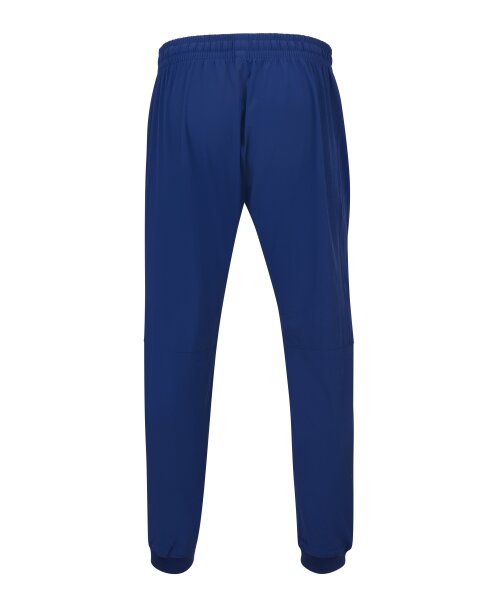This is a detailed stock image showcasing a pair of blue sweatpants set against a stark white background. Visibly empty yet standing upright, the sweatpants exude a sense of casual comfort. The blue hue of the pants is slightly lighter than navy, adding a subtle vibrancy. The image highlights several key features: an elastic waistband that is identifiable by its folds and creases, and cuffs at the bottom of each leg that are a darker shade of blue, likely accentuated by the threading. The sweatpants are long, extending down to the ankles where the fabric becomes tighter. The material appears to be stretchy and comfortable, resembling a typical fleece yet possibly made from a nylon or rayon blend. The pants are seamless in design with no additional patterns or logos, offering a minimalist aesthetic. The clean, white background ensures that all attention remains focused on the well-crafted details of the sweatpants.